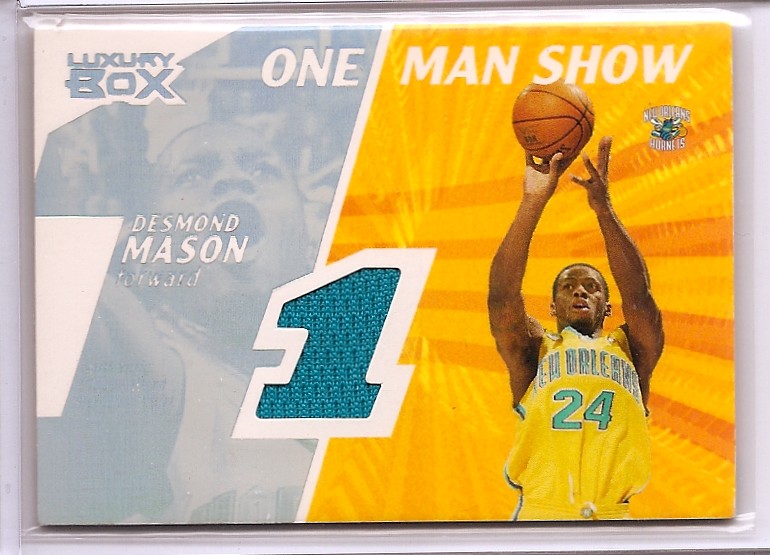This detailed basketball card captures Desmond Mason in a dynamic action shot, prominently featuring him in a mid-air jump, poised to make a play with the basketball in his hands. The color image on the right side of the card shows Mason, labeled faithfully with his number 24 in blue on a vibrant yellow uniform, set against a striking orange background with dark orange streaks. To the left, the card is shaded in light blue, carved into the shape of a number 1 which includes a grayish image of Mason, his mouth open as if calling out or celebrating. Key inscriptions adorn the card: "Luxury Box" on the top left, "Desmond Mason Forward" on the middle left, and "One Man Show" at the top right, which also hosts the New Orleans Hornets logo. Furthermore, there is a hint of an embedded fabric piece, possibly a jersey swatch, sampling the green hue associated with the Hornets’ team colors, making this card not just a visual delight but a collector's treasure.